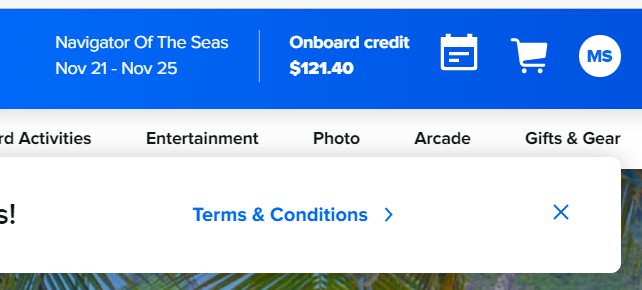"Navigator of the Seas, November 21st-25th: An advertisement highlights an onboard spending card valued at $1.21 with an additional cost of 40 cents. The creative, visually appealing design includes elements such as a calendar, a shopping cart icon, and a circular emblem marked with 'MS.' Activities and entertainment options, including a photo arcade, are showcased, encouraging guests to get some gear. Vibrant imagery features a scenic backdrop of palm trees and lush green leaves against a blue sky, evoking a tropical paradise. The promotional material is neatly presented, with clear terms and conditions, symbolized by a small 'X' for additional information."